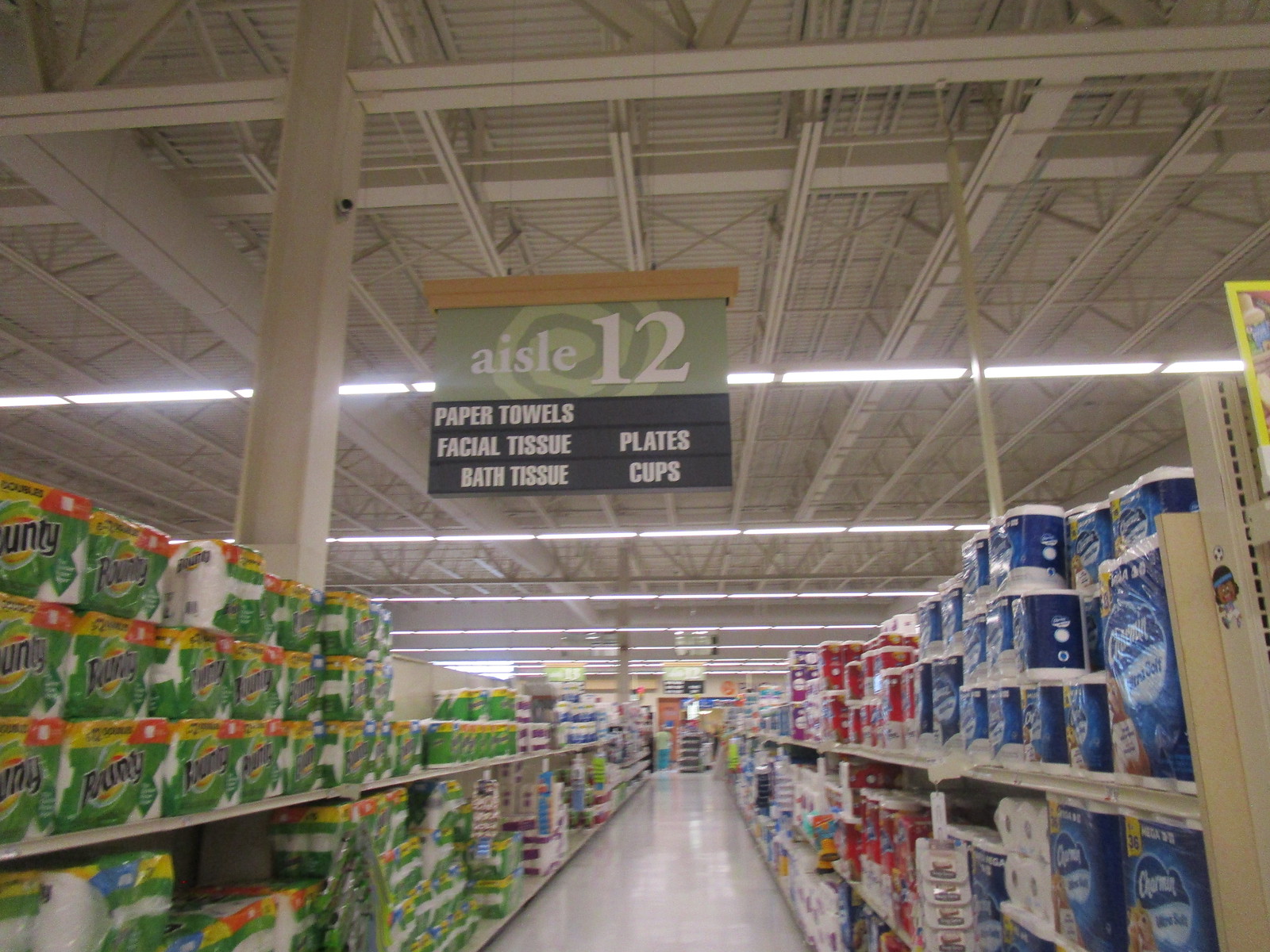This image showcases aisle 12 in a large grocery store, displaying a variety of paper products. Prominently marked with a yellow-framed, green banner, the aisle sign indicates it stocks paper towels, facial tissue, bath tissue, plates, and cups. The store's industrial ceiling, painted white and adorned with exposed beams, spans across the scene. The floor below is white and shiny, reflecting the bright lights from above. To the left, stacks of Bounty paper towels dominate the shelf, while to the right, blue-packaged Cottonelle bath tissues and Charmin products are visible. The aisle extends far into the distance, lined with more paper goods whose brands are indistinguishable in the background. The ceiling's design and lighting suggest this could be a store like Walmart or Kroger.